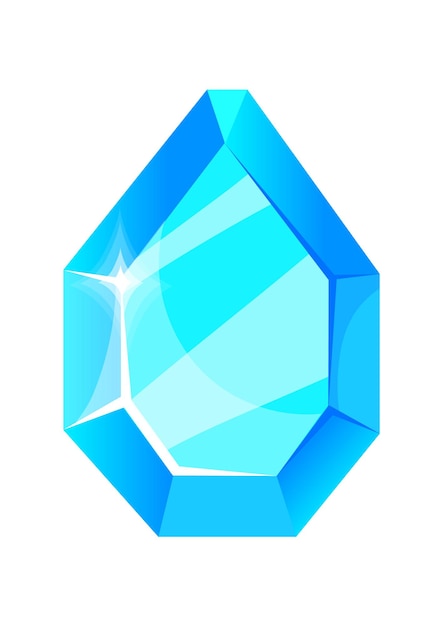The image is a rectangular drawing with its left and right sides being twice as long as its top and bottom. It features a cartoon-like gem and lacks any border or background. This gem is teardrop-shaped with sharp angles, comprising eight sides in total. The gem's design suggests a slope upwards from the sides, making the edges thinner than the center. Predominantly blue, the gem has a dark blue outline, with gradients of lighter blue towards the center, creating a reflective illusion. Various lighter blue lines and diagonal stripes enhance this effect, giving the sense that it's shining in the middle. A distinctive white, four-pointed star on the top left indicates a light flash. The top of the gem is flat. The overall appearance suggests a carved surface, with a combination of V-shapes and square-like facets, possibly evoking an aesthetic from a child’s cartoon, reminiscent of American animation from the 1970s or 80s, or even anime.